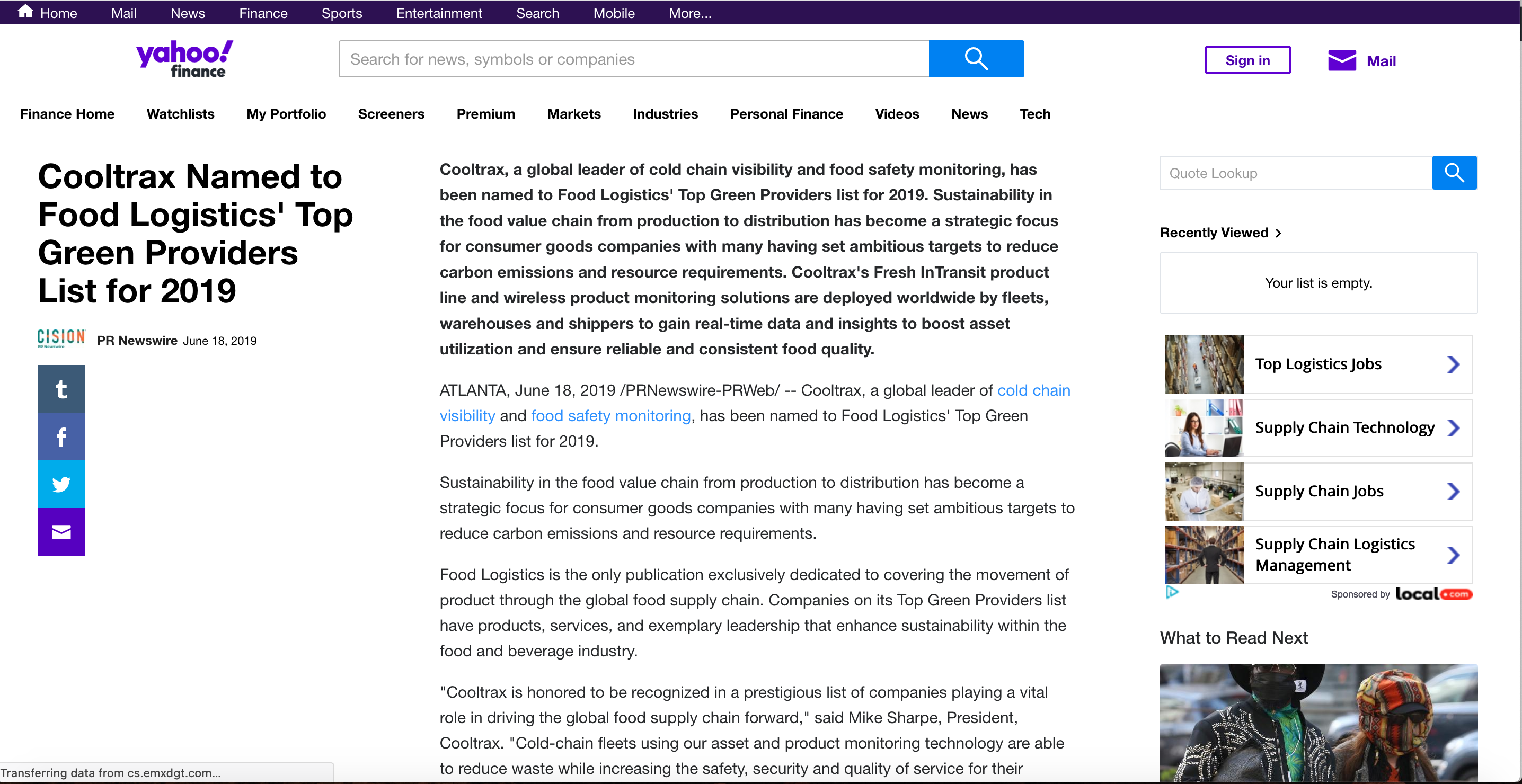The image features a predominantly white background with a detailed interface resembling Yahoo Finance. At the top, a purple navigation bar includes links for Home, Mail, Map, News, Finance, Sports, Entertainment, Search, Mobile, and More. Below this header, larger text reading "Yahoo Finance" is prominently displayed, with "Yahoo" in purple. 

A blue-accented search box sits beside a purple "Sign In" button and a purple mail icon. Directly below, various tabs such as Finance Home, Watchlist, My Portfolio, Screeners, Premium, Markets, Industries, Personal Finance, Visitors, News, and Tech are listed. 

The main content area highlights a headline: "CoolTracks Named to Food Logistics Top Green Providers List for 2019," accompanied by the Cision logo in multiple colors (blue, purple, yellow, and red) and a PR Newswire date stamp of June 18, 2019. 

Social media icons for Twitter, Facebook, and a purple mail icon are positioned at the bottom. The article itself contains three to four paragraphs detailing information about CoolTracks.

To the right, there's an additional search box, followed by a "Recently Viewed" section with a right arrow icon. Below, a list displays thumbnails and blue right-arrow links for "Top Logistic Jobs," "Supply Chain Technology," "Supply Chain Jobs," and "Supply Chain Logistics Management." A "Local" section with a red box and a "What to Read Next" area features an image of two warmly dressed people add further contextual details to the layout.